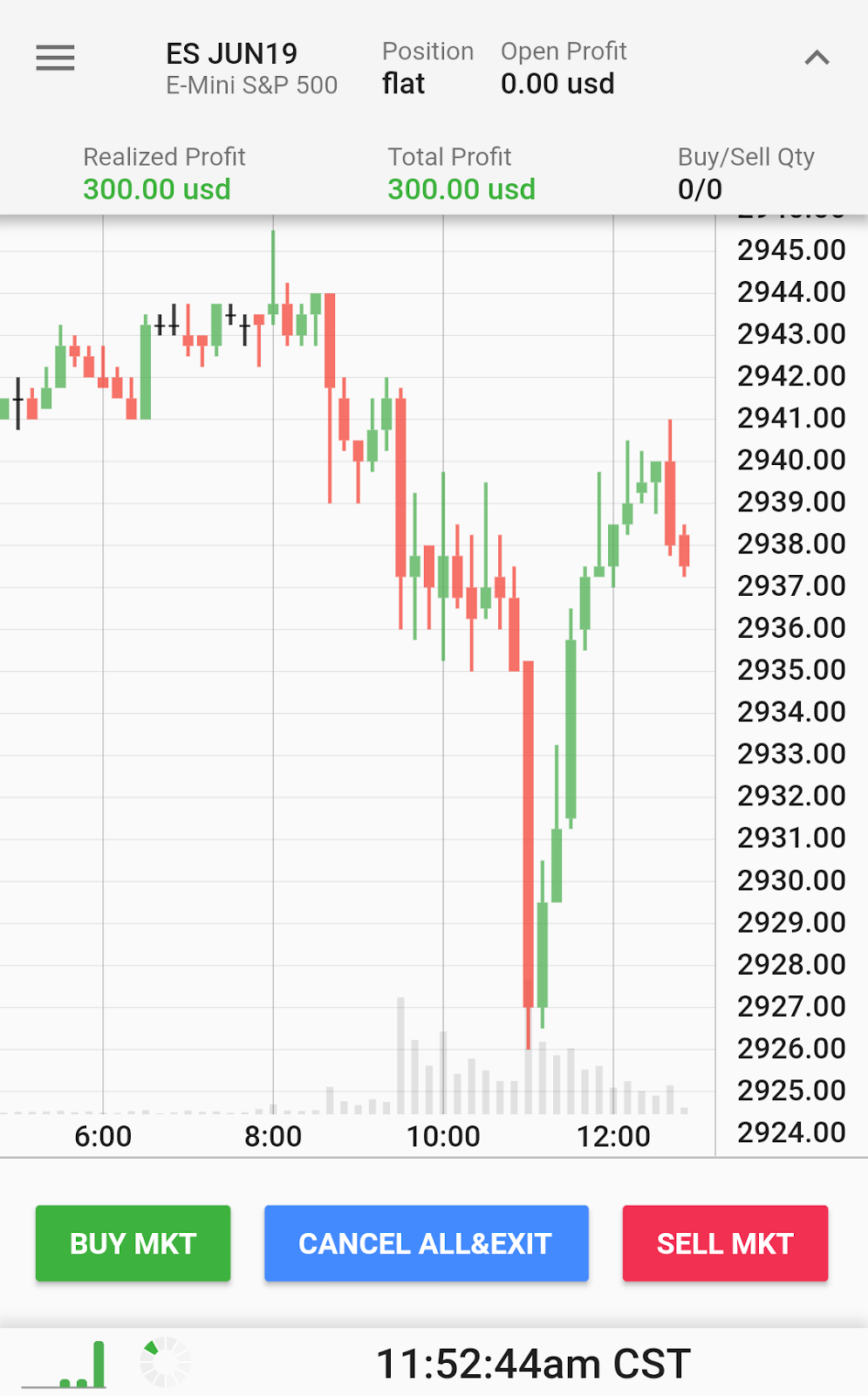The image features a detailed trading dashboard set against a white background. It prominently displays an icon related to E-mini S&P 500 futures. A section labeled "Position" shows a flat, open position with no profit or loss (0.00 USD). The "Realized Profit" for this E-mini S&P 500 trade is listed as 300 USD, bringing the "Total Profit" to 300 USD as well.

Various trading options appear on the dashboard, including indicators for buy/sell quantities (labeled as QT/QTY), with values displayed as 0/0. The chart on the right side shows numerical labels from 2924 to 2945, accompanied by colored rectangles in red, green, and black that mark different points or events on the chart.

A green rectangle features the text "Buy Market (MKT)" in white. Additionally, there is a blue rectangle labeled "Cancel All and Exit" for quick actions, and a red rectangle labeled "Sell Market (MKT)." The timestamp on the dashboard reads 11:52:44 AM CST.

The overall layout of the dashboard combines essential trading metrics, actions, and visual aids to provide a comprehensive trading interface.